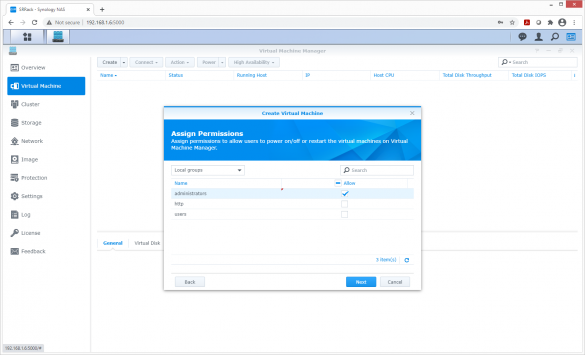The image is a screenshot of a web interface displaying a dialogue box at its center. At the top of the dialogue box, the text, though slightly blurred, appears to read "Create Virtual Machine." Below this header, there is a section titled "Assign Permissions," which seems to provide options for assigning permissions that allow users to interact with virtual machine messages. The content within this section is also somewhat blurry, making the precise wording difficult to discern. The dialogue box features multiple tabs, suggesting the presence of additional settings or options that can be navigated by clicking on these tabs. At the bottom of the dialogue box, there is a prominent blue button labeled "Next" and a white button labeled "Cancel." The overall layout indicates a step-by-step configuration process for setting up a virtual machine.